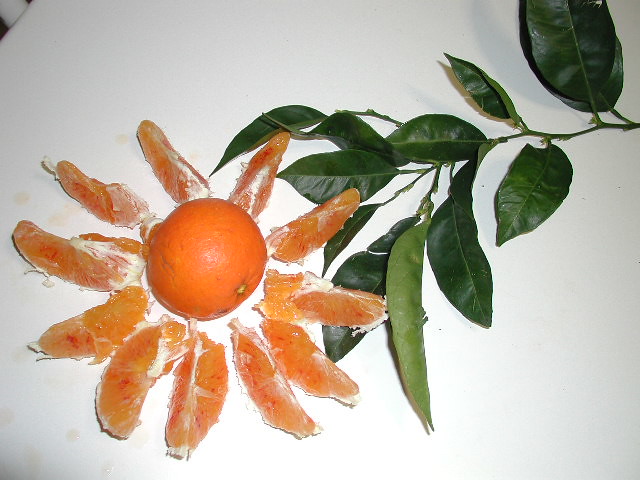This photograph captures a meticulously arranged composition featuring a whole orange resting on a white surface. Surrounding the orange is a radiating circle of peeled orange slices, resembling the petals of a flower or the rays of a sun. The orange slices, with bits of white rind and red flecks still attached, fan out symmetrically from the central fruit. A branch from an orange tree, complete with glossy, dark green leaves, stretches from the right side of the frame towards the left, intersecting with the ring of orange slices. This branch adds a natural element to the arrangement, simulating the appearance of a stem and leaves. The composition is bright, with reflections on the green leaves, and the background remains a clean white, highlighting the vibrant colors of the orange and the leaves. Additionally, a white and black object is partially visible in the top left corner, hinting at a broader setting. The image has a clear, well-lit ambiance, showcasing the detailed textures and colors of the fruit and foliage.